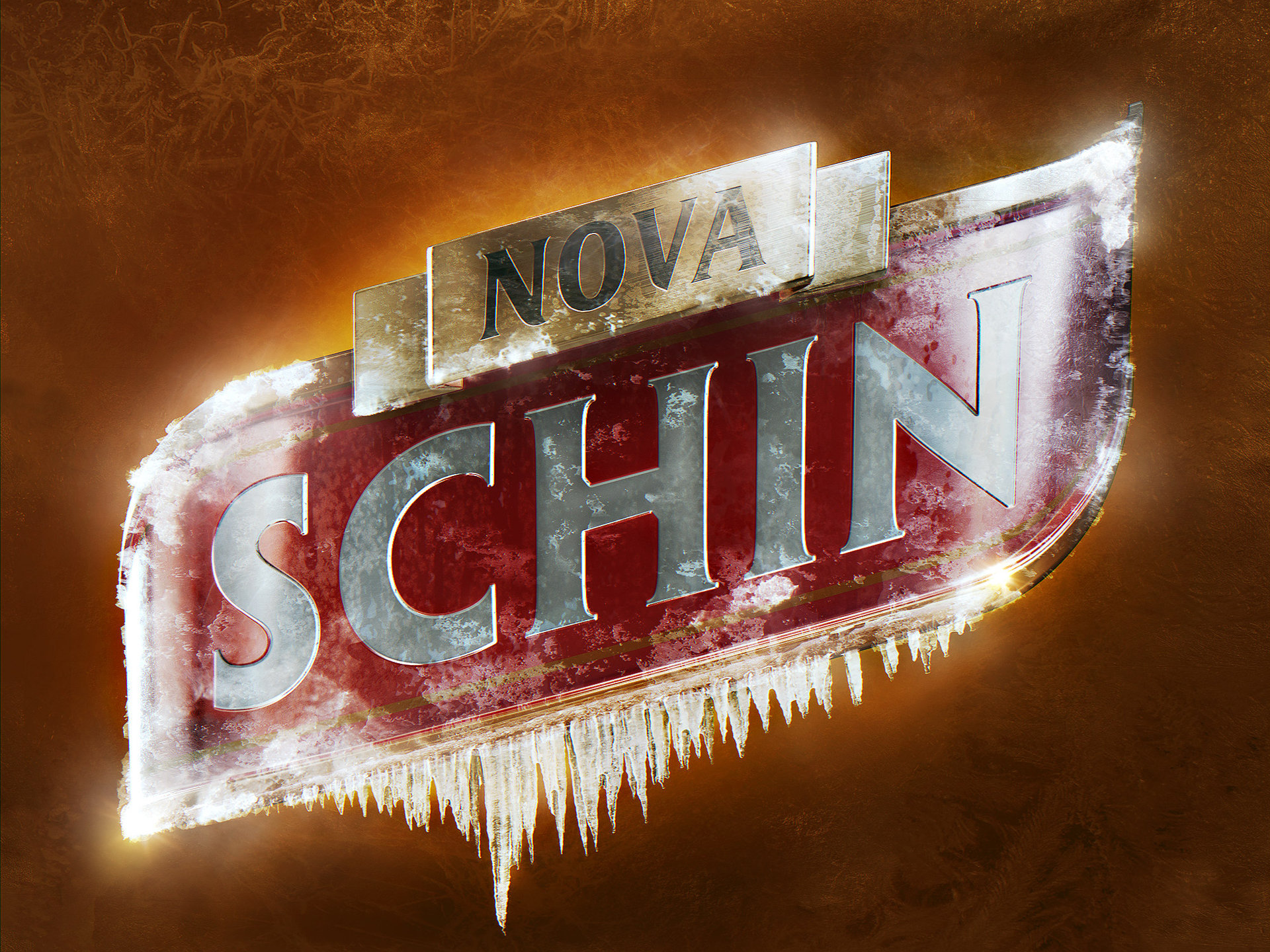This image depicts a sign mounted against a brown background, angled upward to the right at 45 degrees. The sign features two distinct sections: the top section contains the word "NOVA" in black print on a smaller rectangular plaque that mimics the appearance of a ribbon. Below this, the larger main red sign prominently displays the word "SCHIN" in metallic silver capital letters set against a red rectangular background. The red section of the sign curves smoothly, resembling a car's side mirror, especially on the left and right, but tapers off to decorate the sign's bottom with icicles that dangle longest below the letter 'C'. The entire structure is backlit and illuminated, giving it an eye-catching glow. The icy, frosted elements draping the sign suggest it has emerged from a frozen environment, making it reminiscent of promotional material commonly seen in bars, perhaps in an advertisement for beer.